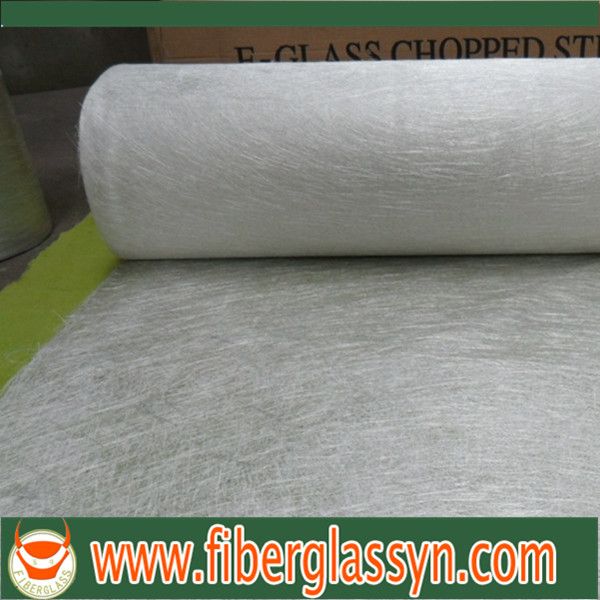The photograph showcases a large, whitish-gray roll of soft fiberglass partially unrolled and placed on a bright green cloth-covered table. Behind the roll is a brown cardboard box with partially obstructed lettering that reads "E-Glass Chopped St." The bottom of the image features a green banner with the website URL, www.fiberglassyn.com, displayed in a mix of red, orange, and white letters. To the left of the URL is a circular symbol with the word "Fiberglass" accompanied by an orange design.